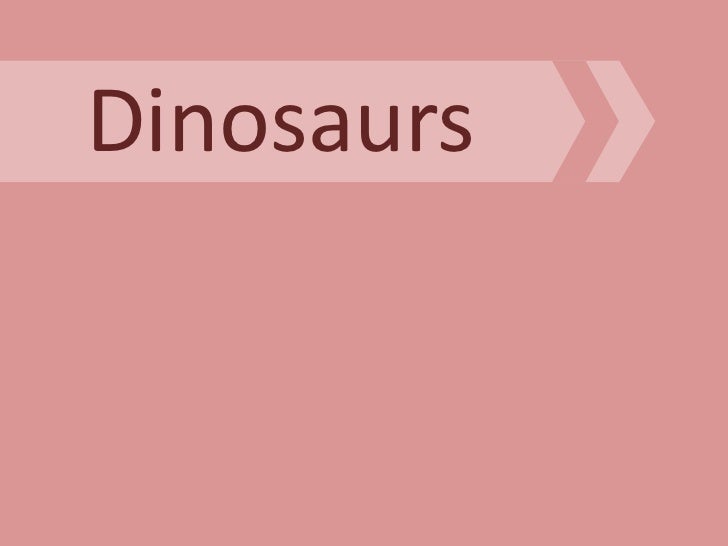The image depicts a square digital slide, resembling a PowerPoint presentation with a light pinkish-tan background. Near the top of the slide, there is a prominent light pink horizontal strip, shaped like a rectangle with a triangular tip on the right side, extending from the left edge and covering approximately 70% of the slide's width. Above this strip, there is another horizontal strip also shaped like a rectangle. Centered within the lower strip, written in dark brown text, is the word "Dinosaurs," with the capital "D" and lowercase letters for the rest. Above and parallel to this strip is a smaller, similar horizontal strip, also pointing to the right.